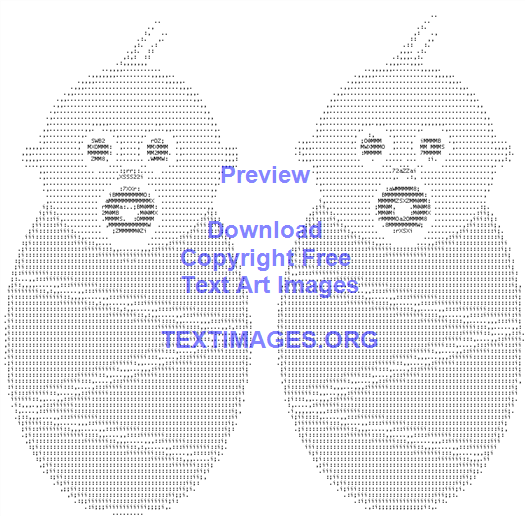This image features an intricate text art depiction of two identical swaddled babies with minimal hair—each with just a couple of strings on their bald heads—and pacifiers in their mouths. The entire illustration is composed meticulously of various letters, numbers, and symbols set against a blank white background. Both babies are tightly wrapped in blankets, their round heads and open eyes clearly defined by the detailed text characters. Prominently displayed in blue text at the center, overlaying the text art, is the message: "Preview, download, copyright-free text art images" followed by the website address, textimages.org. The careful arrangement of the text elements culminates in an eye-catching and cohesive artwork that captures the whimsical yet impressive potential of text art.